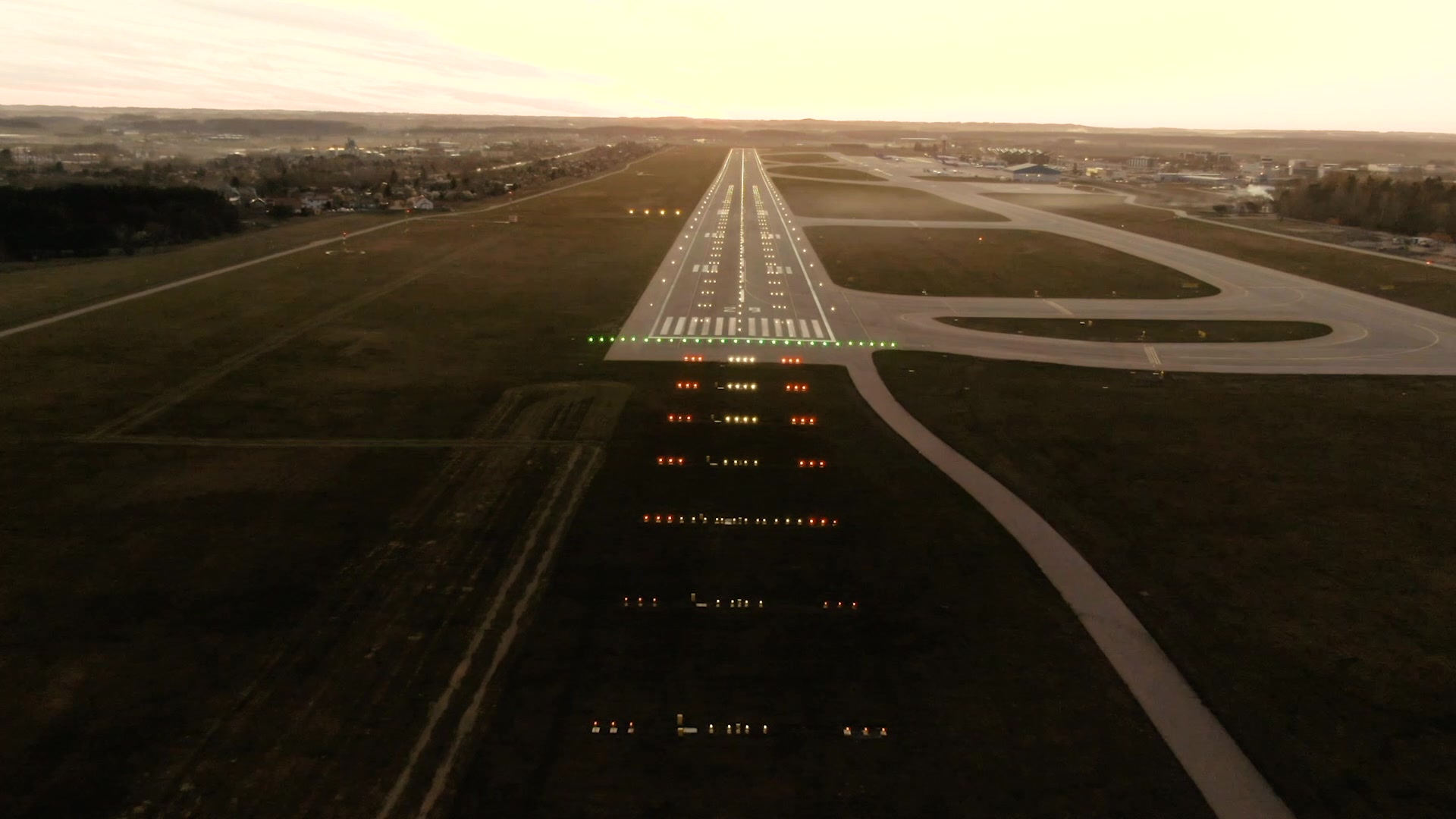The image depicts an airport runway from the perspective of an approaching airplane. The runway is aligned dead straight ahead, adorned with numerous white markings and various colored lights. At the beginning of the runway, green lights indicate where to start landing. Further down, red and yellow lights signal different stages of the approach and slowing down. Just before the runway, horizontal lines with integrated lights and vertical lines listing numbers are visible. Off to the left, there is a dark-colored grass field, though it's likely green under different lighting or weather conditions. On the right side, a network of winding roadways leads away from the runway, facilitating the aircraft's transition to the airport. This side also features additional grass fields. The far distance reveals a tree line, and scattered buildings and trees dot the surroundings. The overall scene is dimly lit, indicating a possible overcast day with a bright but clouded sky, especially clear in the upper left-hand corner of the image.